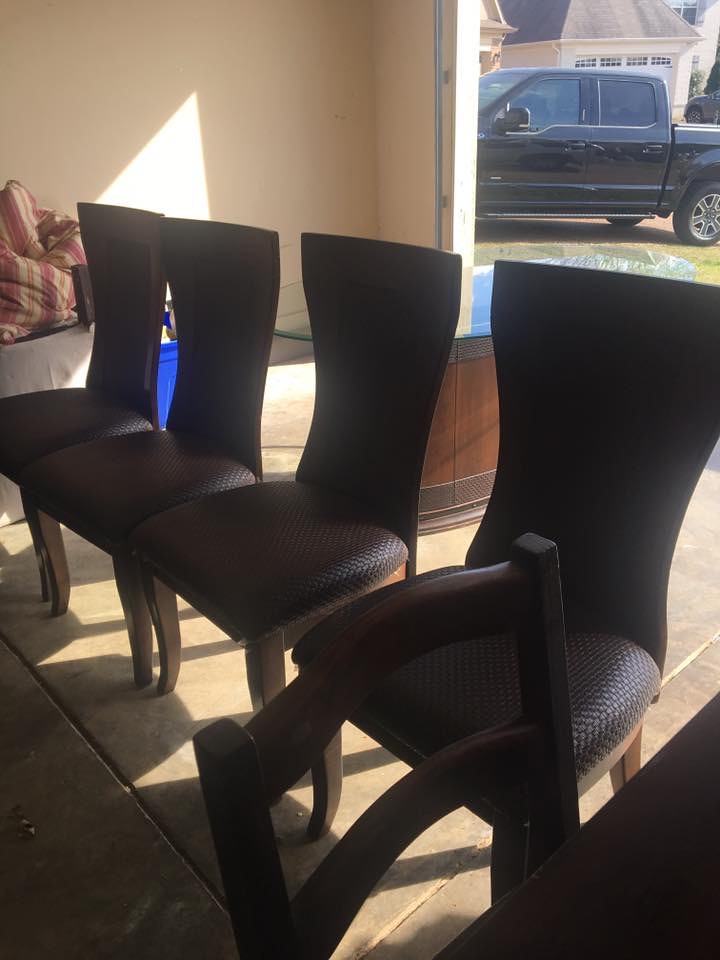This detailed photograph vividly captures the inside of a garage with a cement floor and an open garage door letting in sunlight. In the foreground, there are five high-back chairs, predominantly black with padded seats and wooden, mahogany-toned legs. Four of these chairs are aligned, facing the camera, allowing a clear view of the black seats and solid black chair backs. The fifth chair, differing slightly with two horizontal wooden slats on its back, is positioned near what appears to be an oval glass table featuring a solid mahogany base.

The off-white walls of the garage are discernible in the background, with some wood and possibly paper bags scattered towards the rear, hinting at typical garage storage or yard waste. The strong sunlight streaming through the open garage door causes the chair legs to cast visible shadows on the cement floor, highlighting the time of day.

Outside, the photo captures a black super duty cab truck parked in the driveway, partially revealing portions of the neighboring lawn. Beyond the driveway, an off-white or tan-colored house with black tiles is visible, contributing to this scene’s overall suburban setting.